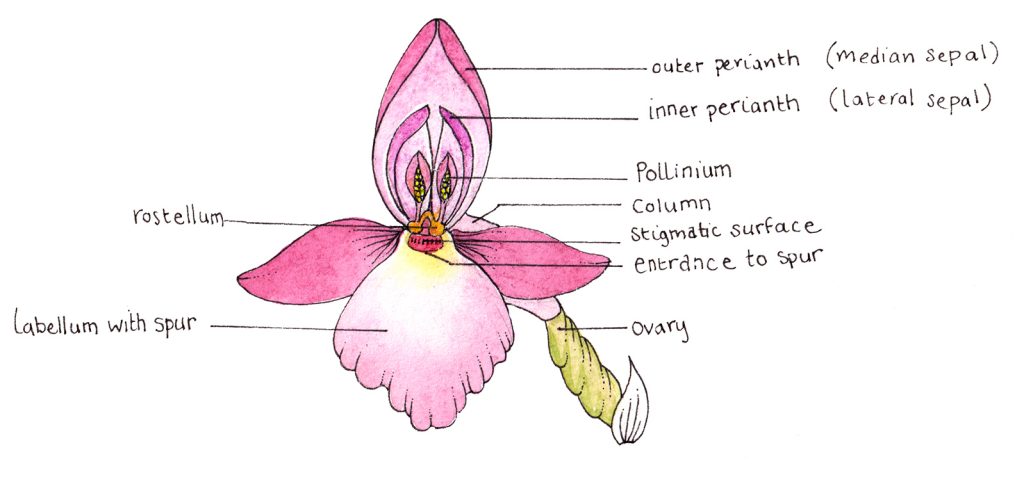A detailed pencil drawing of a pink orchid flower, resembling a student's anatomy diagram for a science project, is the focal point. The flower's parts are meticulously labeled with black pencil text on a white background. From the top, the outermost petal, labeled "outer perianth" with "median sepal" in parentheses, stands upright. Inside this petal, there are additional elements labeled "inner perianth" with "lateral sepal" in parentheses, featuring various shades of pink and yellow. Below this, shorter protrusions marked "pollinium" are visible. The central part of the flower includes a labeled "column," leading down to the "stigmatic surface" and the "entrance to spur." The lower petal, depicted protruding outward, is labeled "labellum with spur," while a line points towards the middle, identifying the "rostellum." The stem, extending to the right and labeled "ovary," anchors the flower. This detailed illustration shows each part connected by lines to its respective label.